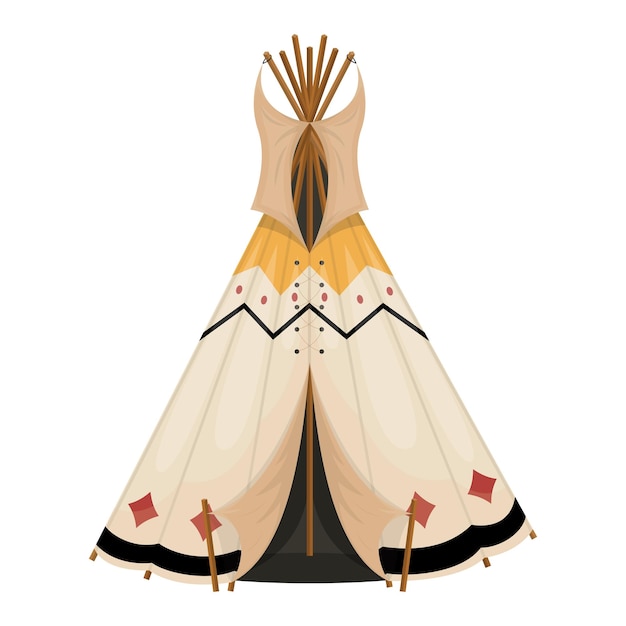The image features a detailed drawing of a Native American tipi with a white background. The tipi is constructed from a wooden frame consisting of seven visible poles that extend through the top for venting. The structure is primarily white, adorned with a mix of yellow, red, black, and blue colors in various patterns. 

At the very top, yellow zigzag patterns interspersed with red dots are present, followed by a black zigzag pattern below. Moving downward, the design incorporates red diamond accents on the lower portion, coupled with a thick black stripe encircling the base. The tipi flares out wide at the bottom, much like a dress, with a waistline tapering the structure from top to bottom. 

The entrance of the tipi is propped open with sticks on each side, offering a glimpse into the interior. The overall appearance, combining the shape and decorative elements, gives it a visual resemblance to a dress hung on a frame or possibly designed to mimic the look of a dress.